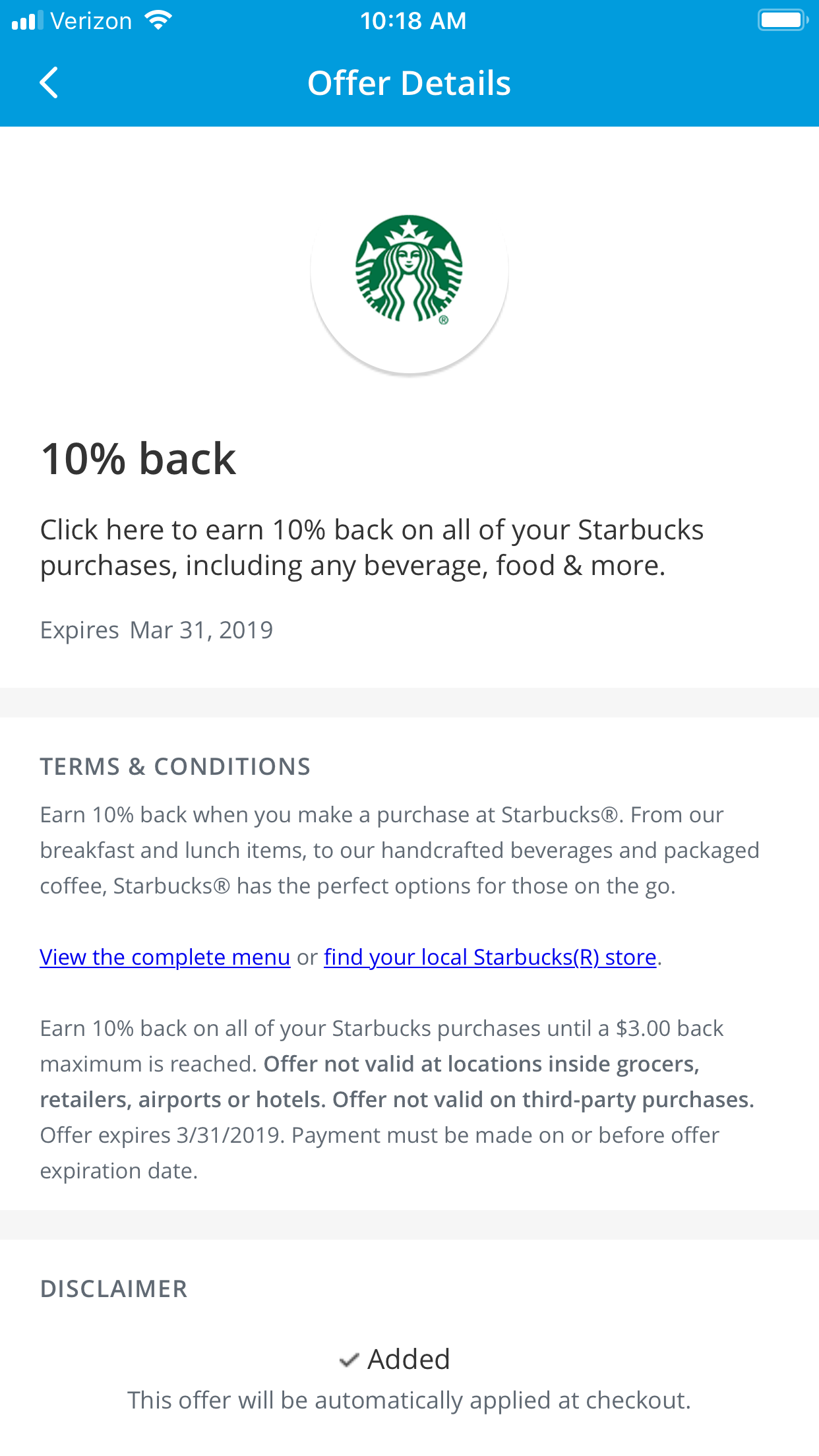The image on the website is primarily text-focused, set against a clean white background. At the top, there is a blue bar on the upper left indicating "Verizon," alongside the center time display reading "10:18 a.m.," and a full battery icon positioned on the upper right. Below this header, centrally aligned and in white text, is the headline "Offer Details."

Dominating the central portion of the page is the iconic Starbucks logo, which features a white circle encasing a green circle with the classic image of the Starbucks siren in white.

Below the logo, text announces a promotional offer stating, "Click here to earn 10% back on all of your Starbucks purchases, including any beverages, food, and more. Expires March 31st, 2019." Following this, a smaller section reads "Terms and Conditions," presented in a straightforward blue font.

Beneath this, the page provides further engagement options in blue text, inviting viewers to "View the complete menu" or "Find your local Starbucks store." Additional details clarify that customers can earn 10% back after a minimum spend of three dollars, with specifics on where the offer is applicable. A white line separates this section from the rest of the content.

Toward the bottom of the image, there is a note labelled "Disclaimer," centered with a checkmark, stating, "Added." The final piece of information indicates that "This offer will be automatically applied at checkout."